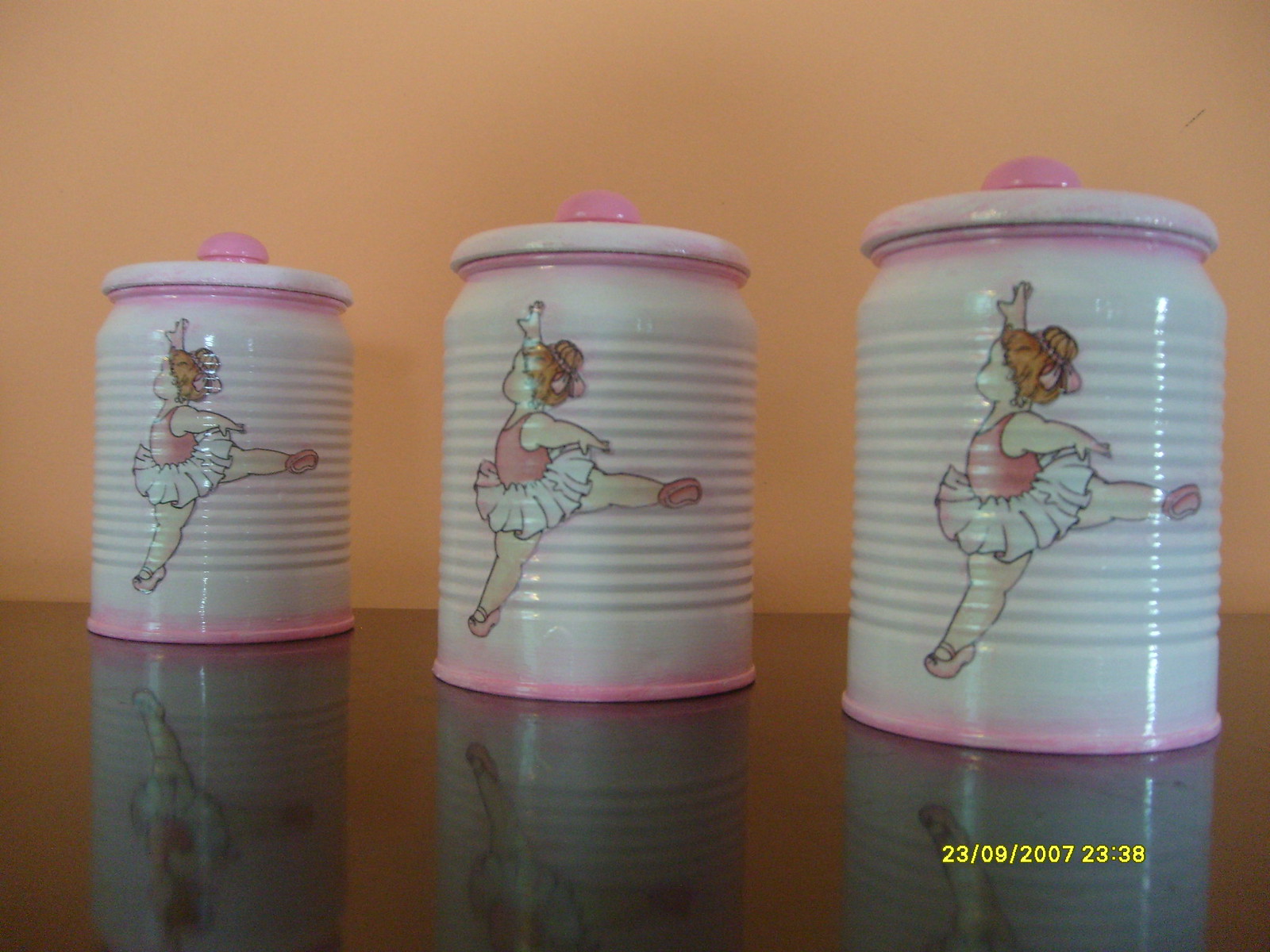This indoor color photograph, seemingly taken on September 23, 2007, at 23:38, depicts three identical ceramic cookie jars. Each white porcelain jar features pink rims and round pink handles on top. Adorning the front of the jars is a chubby young ballerina girl, dressed in a pink top and white tutu, her hair elegantly pulled into a bun. She is captured in mid-air performing a plié, with her right arm reaching straight up and her left arm extended gracefully to the side. Though the profile of her face is visible, its details remain indistinct. The jars rest on a reflective dark surface, possibly a black table, contrasting with the orange-peach colored wall in the background. The lower right-hand corner of the image contains a yellow date stamp reading "2309-2007" along with the timestamp "2338". No other text or print is present, suggesting the photograph might have been taken to market these items online.